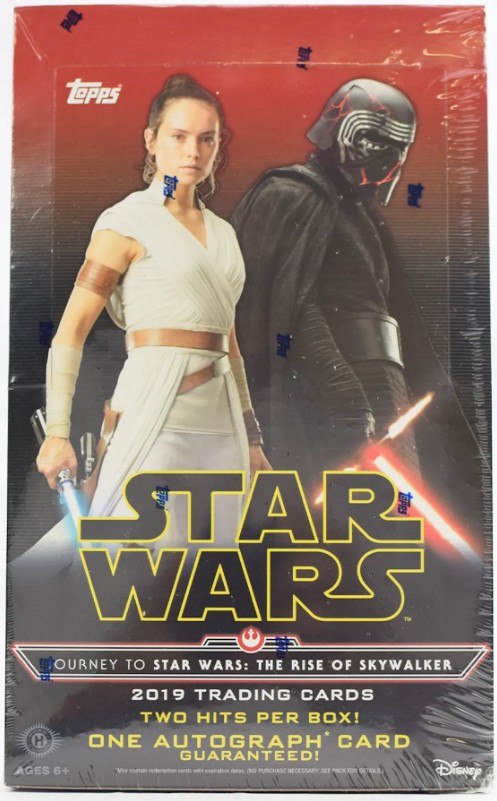The image depicts a collectible trading card encased in plastic, branded with the TOPS logo in small, white text at the top left corner. The background seamlessly transitions from red at the top to black at the bottom. The card prominently features two characters: on the left, a woman in a white robe with a brown band around her waist and arm, wielding a blue lightsaber; and on the right, a figure resembling Darth Vader, dressed in an all-black outfit complete with a black helmet, cape, and gloves, and holding a red lightsaber. Positioned centrally on the card, the text reads "STAR WARS" with gold trim, followed by "Journey to Star Wars: The Rise of Skywalker." Below this, it specifies "2019 Trading Cards," along with the promises of "Two Hits per Box" and "One Autograph Card Guaranteed." The Disney logo is visible in the bottom right corner and an age restriction of "6+" is noted in the bottom left corner.